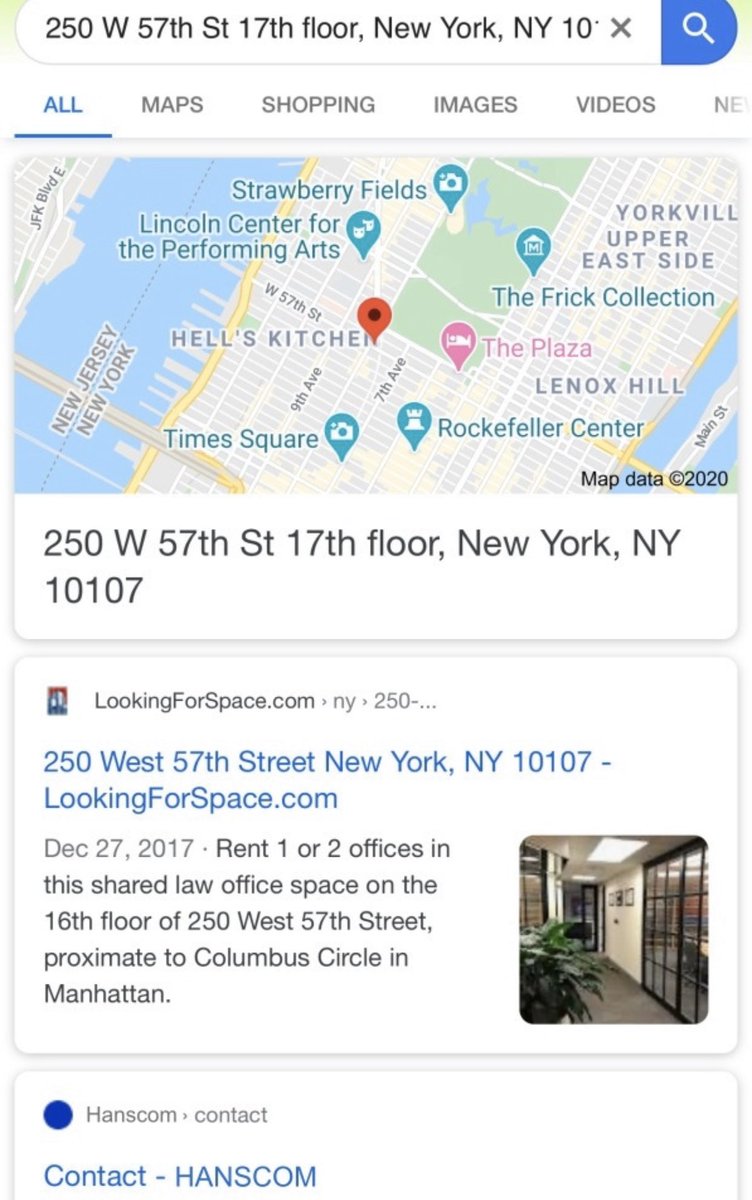This image displays a website interface spotlighting office space details in Manhattan. The search bar at the top contains the address "250 West 57th Street, 17th floor, New York, New York," with a blue search icon beside it. While the zip code is incomplete, the search bar's text is highlighted in blue and underlined.

Directly below the search bar, a map of a part of Manhattan is visible, featuring pins indicating notable locations such as Times Square, Rockefeller Center, and various dining spots. Under the map, the address "250 West 57th Street, New York, New York" is reiterated.

The section beneath contains a white square box with text reading "lookingforspace.com, New York, from 250 West 57th Street, New York, New York, 10107," with the web address "lookingforspace.com" highlighted in blue. The date "December 27, 2017" follows, with details about leasing one or two offices in a shared law office space located on the 16th floor of the same building, near Columbus Circle in Manhattan. An image of the office space with a plant is also embedded within this section.

Below this information, another square box is labeled "Hanson Contact," with the contact email "contacthanscon, H-A-N-S-C-O-N, Hanscom" noted. A prominent blue dot is situated in the upper left corner of this box, and part of the website text is cut off, fading into the background.